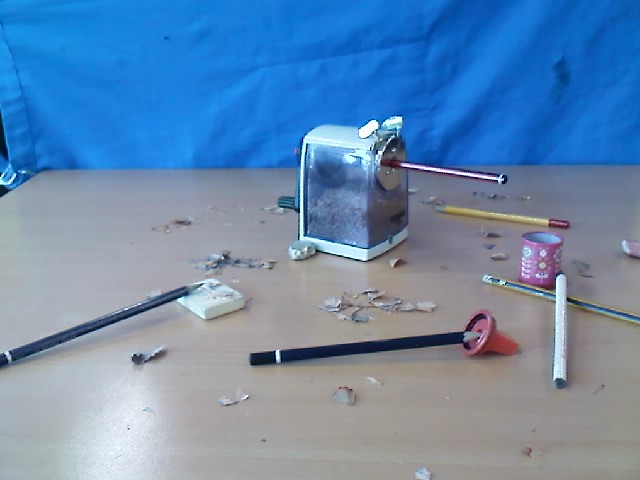The photograph captures a detailed scene centered around a wooden table set against a blue fabric backdrop, possibly a tarp. Dominating the middle of the table is an old-fashioned, crank-powered pencil sharpener with a white exterior and a clear body, revealing accumulated pencil shavings inside. A brown pencil is actively being sharpened in it, surrounded by loose pencil shavings scattered across the table. Beside the sharpener, a yellow pencil rests on the tabletop. Towards the lower left of the image, a black pencil lays diagonally, its lead tip supported by a square eraser. On the table's right side, a white pencil lies crossed over a black pencil next to some pink tape. Additionally, a broken eraser piece and a small plastic pencil sharpener can be seen among the drawing pencils and shavings, conjuring a scene reminiscent of a busy school desk.